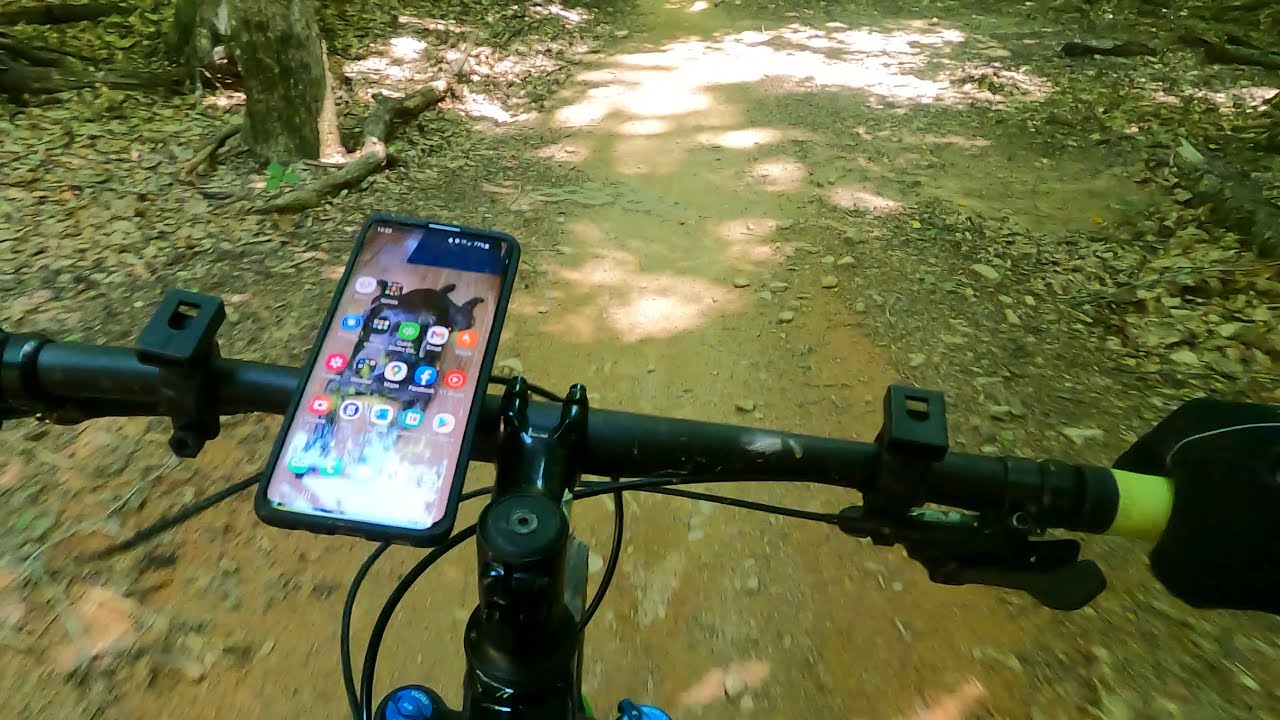The photo captures the view from a bicyclist's perspective, showcasing the long, flat, black handlebars of the bike held on the right side by a gloved hand wearing a black glove with a neon yellow grip. Mounted on the left side of the handlebars is a smartphone, partially obscured by a sunbeam. Despite the glare, some icons are identifiable, including Facebook, Gallery, Camera, Gmail, and Google Maps. The background reveals a dirt path strewn with rocks and green, mossy patches, lined with dead leaves and tree stumps. The scene is dappled with sunlight filtering through the trees, casting bright splotches of light on the trail ahead.